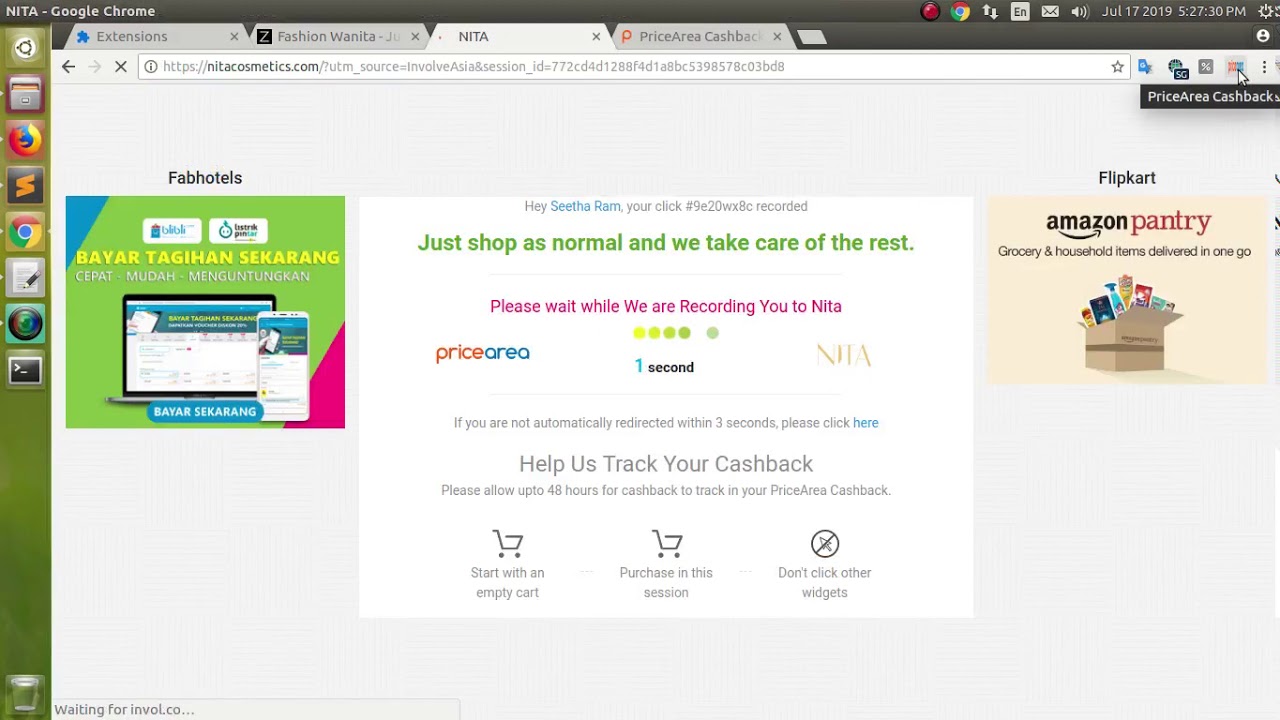This screenshot depicts a detailed view of a desktop interface actively using the Google Chrome browser. At the top, a black banner displays "NITA" alongside "Google Chrome" in white text. To the far right of this banner, several icons are visible: a red dot, a Google icon, uploading and downloading status, an "EN" language indicator, an email icon, a sound icon, and the current time and date.

On the left side of the screen, a vertical sidebar features a series of icons, including those for Firefox and Google, among others, with a trash can icon situated at the bottom left. 

In the browser window, several tabs are open:
1. Extensions
2. Fashion Juanita
3. NITA (currently active)
4. Price Arena Cashback

The active tab, titled "NITA," displays a search bar with the website address, alongside various advertisements:
- A small square ad for Fab Hotels on the left.
- A central banner with a generic cashback icon.
- An ad for Amazon Pantry.

Additionally, a notification reads "Please Wait While We Are Recording You To NITA," suggesting an ongoing process or recording activity related to the NITA website.